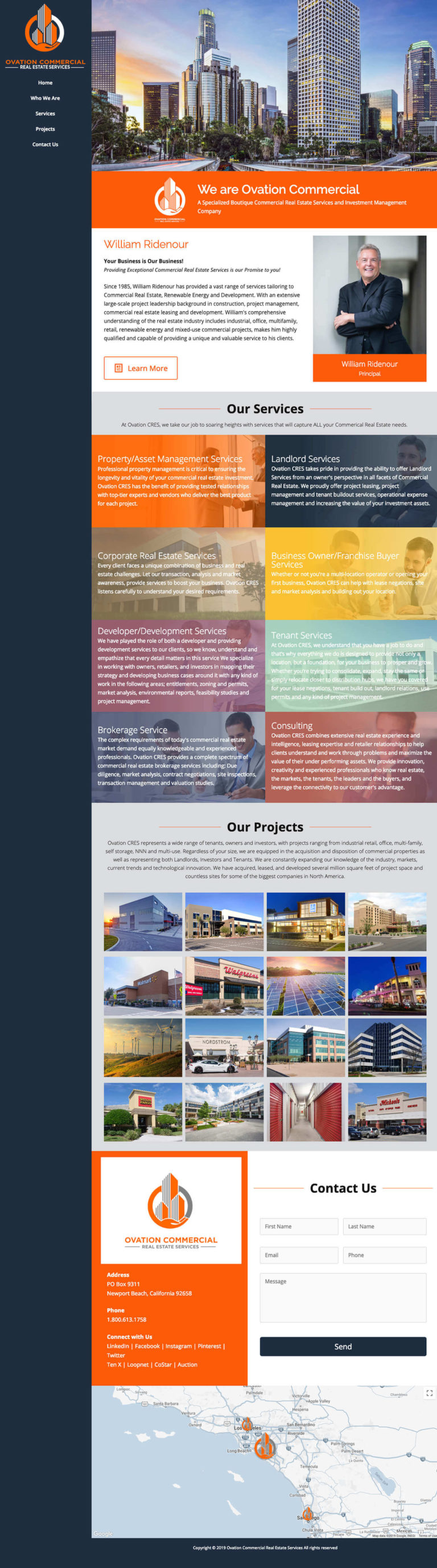This screenshot captures a detailed view of a business website. At the top, a large banner image showcases a stunning city skyline filled with skyscrapers. Directly beneath the banner, there is a professional photo of a man dressed in a dark black suit. He is smiling with his arms crossed and looking directly at the viewer. The text next to his image identifies him as William Renador and provides a brief description of his role or credentials. Below this introduction, the website lists four categories of services that the company offers. Further down, there is a section titled "Our Projects," which includes a short description and a grid of 16 images depicting various large buildings. In the bottom right corner of the screen, there is a "Contact Us" section. At the very bottom of the screenshot, a map of a coastal region is displayed, although it does not clearly indicate the company's location. This screenshot provides a comprehensive overview of the website's key elements.